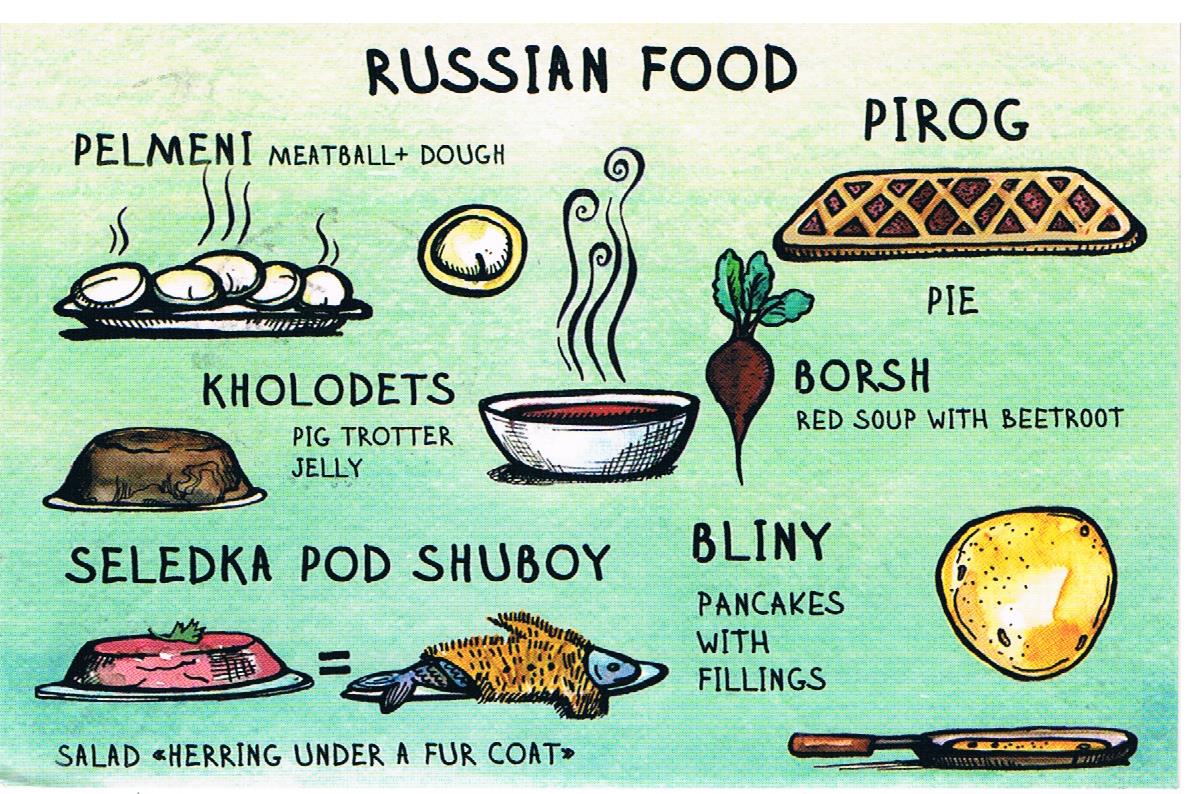The image is an illustrative drawing showcasing a variety of traditional Russian foods against a gradient background that transitions from green to yellow. At the top center of the image, in bold black font, it reads "Russian food." Each item is depicted with a corresponding cartoonish drawing along with its Russian name and a brief English description:

- Top left: **Pelmeni (meatball plus dough)** - Illustrated as white, circular dumplings with steam rising from them, served on a plate.
- Below Pelmeni: **Kolodets (pig trotter jelly)** - Shown as a brown, gelatinous mold resembling Jell-O, placed on a dish.
- Below Kolodets: **Seledka pod shuboi (salad herring under a fur coat)** - Depicted as a blue fish wearing a brown fur coat, suggesting a layered salad with herring.
- Center: **Borscht (red soup with beetroot)** - A bowl of steaming red soup, garnished with a drawing of a beet with green leaves.
- Top right: **Pirog (pie)** - A rectangular pie illustrated with layers of brown and red, possibly resembling a lasagna.
- Below Borscht: **Blini (pancakes with filling)** - Shown as yellow circular pancakes, one in a silver frying pan with a brown handle.

Each dish is meticulously labeled, combining colorful and playful artwork with concise English translations to provide a clear and engaging representation of the various Russian culinary delights.